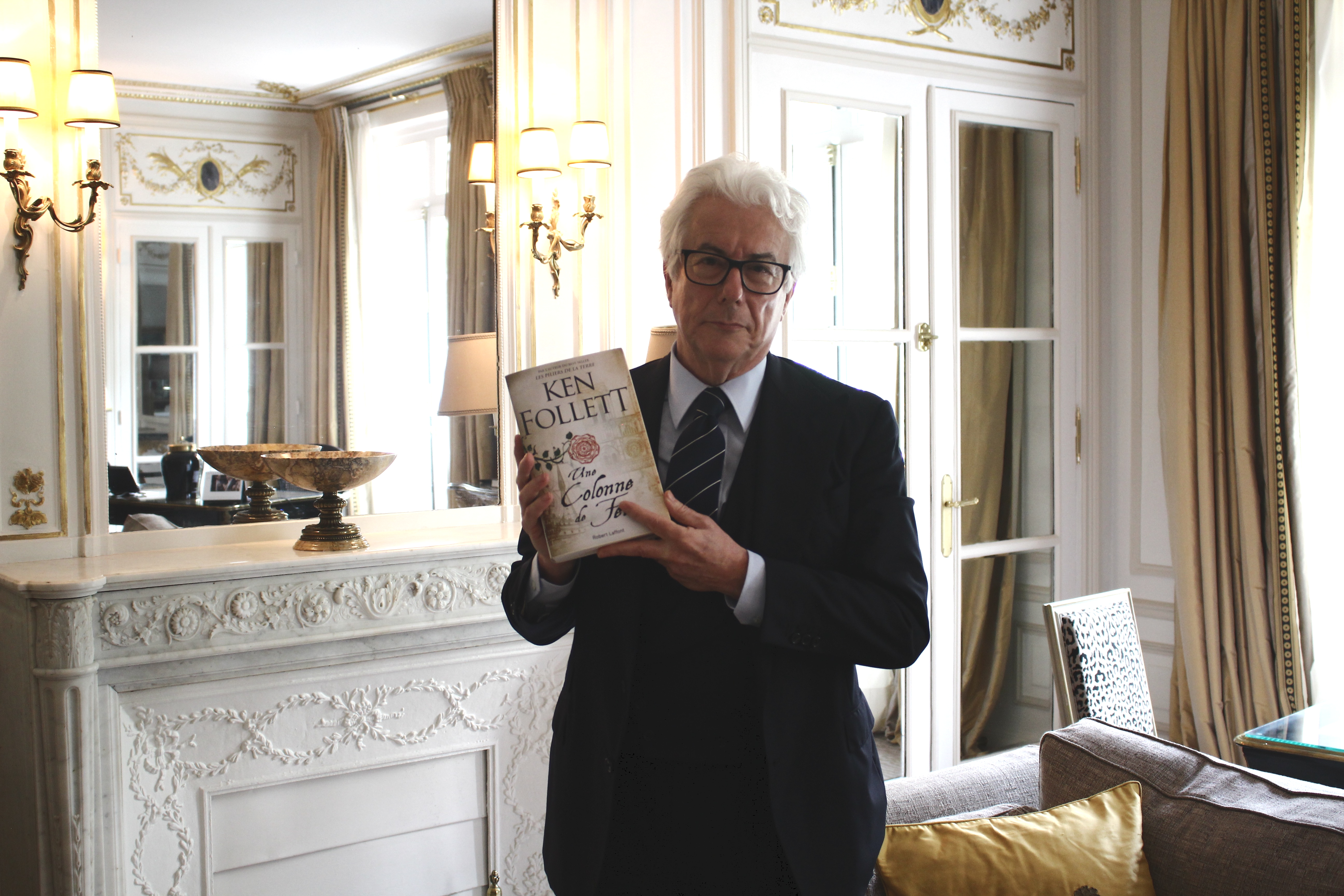In this photograph, author Ken Follett is standing in an elegantly furnished room, showcasing a French edition of one of his novels, likely "A Column of Fire." The book, featuring a white and brown cover with a pink flower, is held with both hands to his left side. Follett, a white male with short white hair, sports thick black-rimmed glasses, a black suit jacket, a white undershirt, and a dark tie adorned with white stripes. The room exudes luxury, with a finely detailed interior that includes an intricately engraved white fireplace topped by a large mirror, flanked by ornate light fixtures. In front of the mirror sits a decorative bowl. The background also reveals polished woodwork, a double glass door, a table with a chair, a couch with a pillow, and a doorway.